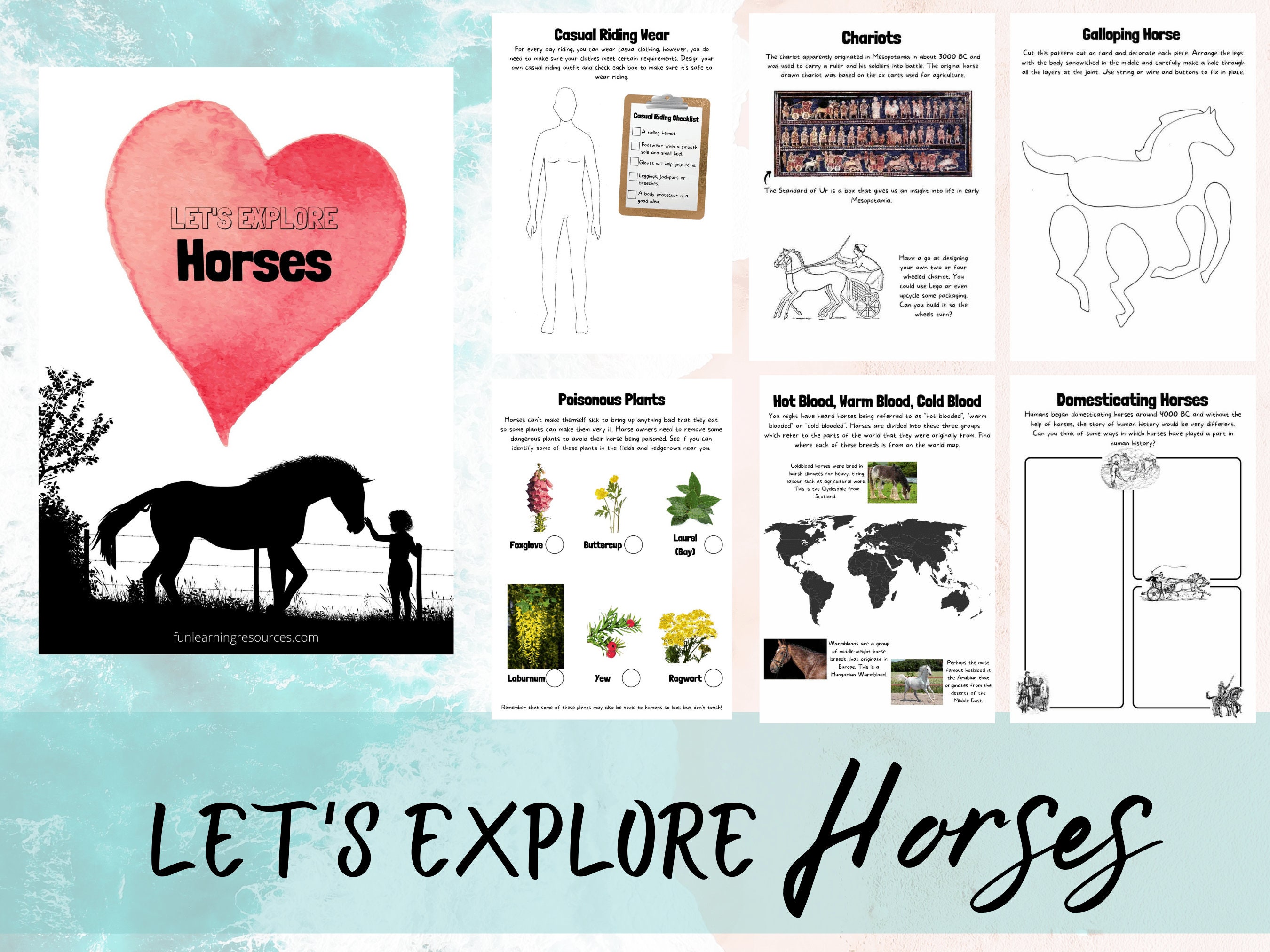This image appears to be an educational pamphlet from funlearningresources.com titled "Let's Explore Horses." The picture prominently features a large heart containing a silhouette of a horse with a little girl petting it, set against a backdrop with a barbed wire fence and grassy field. This heart image is captioned with "Let's Explore Horses," and there's also the website funlearningresources.com printed in white letters at the bottom.

The right side of the pamphlet contains six informative sections: 

1. **Casual Riding Wear** - This section includes an outline of a human figure and presumably details what casual riding attire one should wear, featuring checkboxes and illustrations.
   
2. **Chariots** - Illustrates the historical use of horses in chariot riding, showing images from ancient Rome and Egypt, with riders and horses depicted pulling chariots.

3. **Galloping Horse** - Shows the anatomy of a horse and provides cut-apart pieces to assemble a galloping horse model, illustrating movements of different parts like the torso, head, tail, and legs.

4. **Poisonous Plants** - Highlights various flora that are toxic to horses, featuring images like red flowers, yellow buttercups, green laurel leaves, and red berries.

5. **Hot Blood, Warm Blood, Cold Blood** - Explains the different types of horse temperaments and origins, with illustrations of different horse breeds and a world map.

6. **Domesticating Horses** - Depicts historical scenes of horses being domesticated, used in various capacities such as knights on horseback and noblemen.

Encased in a light blue border, the pamphlet serves as a detailed, interactive guide aiming to educate readers, particularly children, about the world of horses in an engaging manner.